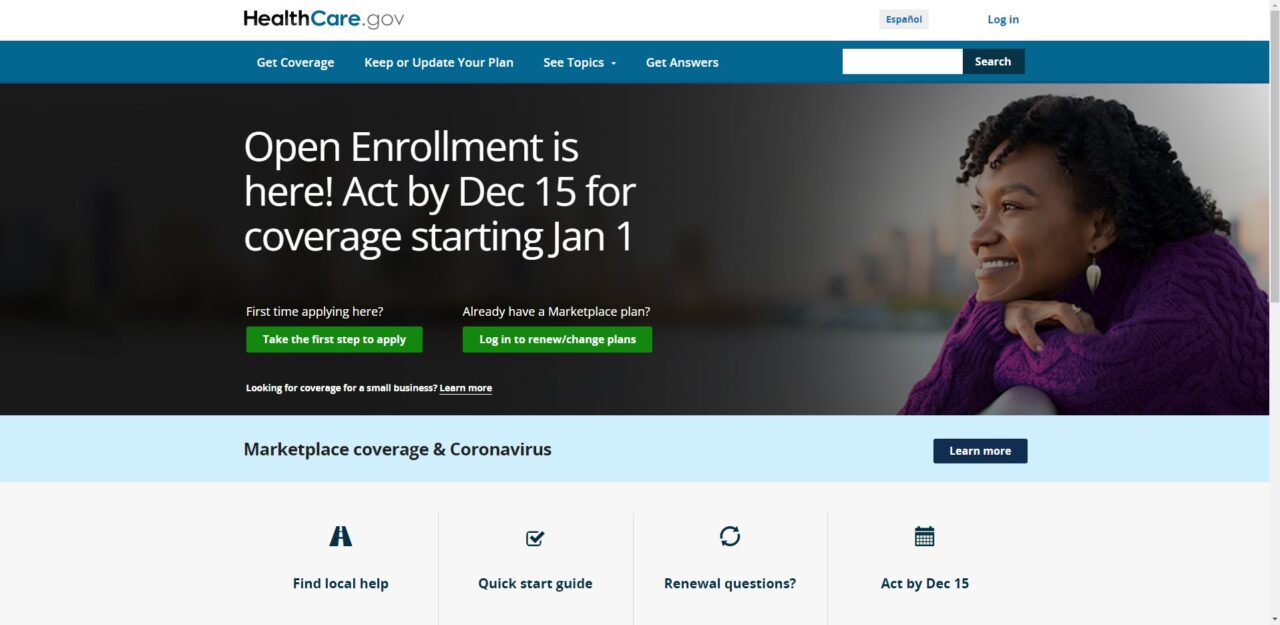The image is a detailed screenshot from the healthcare.gov website, showcasing a neatly organized layout for users seeking health coverage information. The site's header features the healthcare.gov logo, with "Health" in black lettering, "care" in a greenish-blue hue, and ".gov" in gray, all set against a white background. To the right, there is a Spanish translation button with a light gray background and blue text, alongside a plain white login button also in blue text.

Beneath the header, a long rectangular menu bar is displayed, offering clickable links in white text, listing options such as "Get Coverage," "Keep or Update Your Plan," "See Topics," and "Get Answers." Adjacent to the menu bar, a search bar with a white background and a dark blue search button labeled "Search" in white text allows users to quickly find specific information.

A prominent part of the page features an image of a woman with short black hair, donning a purple sweater, seated against a cityscape background. To her left, white text announces critical information: "Open Enrollment is Here. Act by December 15th for coverage starting January 1st." Directly underneath this announcement are two green rectangular buttons.

At the bottom of the page, a light gray background contains additional helpful resources, displayed as icons and text. These options include "Find Local Help," "Quick Start Guide," "Renewal Questions," and another reminder to "Act by December 15th."

Overall, the webpage presents essential health coverage information in an accessible and visually appealing manner, using a combination of text, buttons, and images to guide users through the enrollment process.